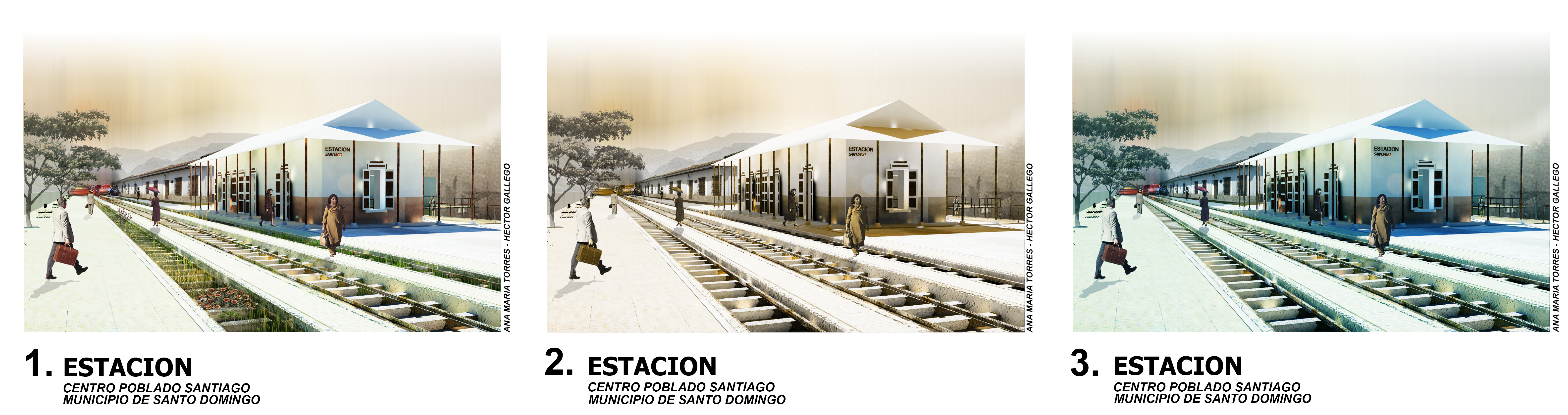The image comprises three distinct visuals, each showcasing a railway station identified as Estación 1, Estación 2, and Estación 3, with accompanying Spanish text "Estacion Centro Poblado Santiago Municipio de Santo Domingo." The artwork reflects a transition through different times of the day, evident from the varying sky colors that range from light orange in Estación 1, to darker brown in Estación 2, and light blue in Estación 3. Each visual consistently features people walking and waiting on the platforms beside the tracks, underscored by a digitally generated aesthetic. The buildings stand predominantly white, adorned with distinct trim colors—blue in one, brown in another. The background subtly includes a tree and some hills under a poorly lit sky. Artist’s names, "Anna Maria Torres" and "Hector Galego," are inscribed along the borders of each image, enhancing the cohesive yet diverse portrayal of this tranquil, small-town railway scene.